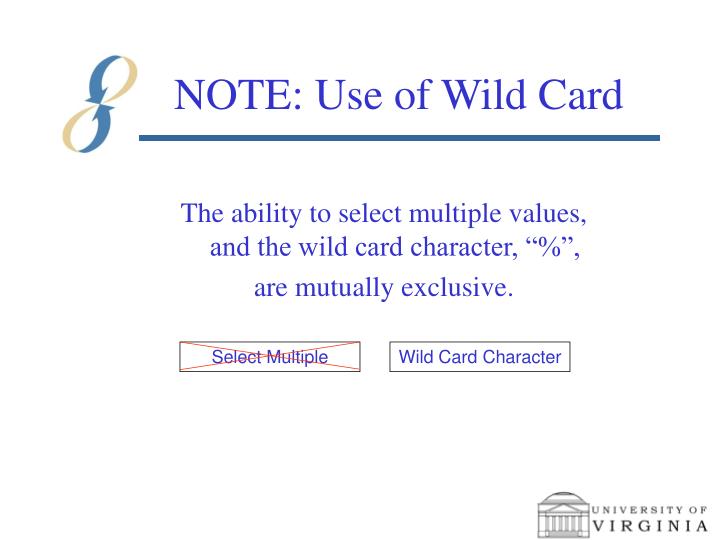The image is an infographic with a white background, presented in a landscape orientation. At the very top, the headline reads "NOTE: USE OF WILDCARD" in dark purple, all-uppercase text. Below this headline is a horizontal dark teal line. To the left of the headline, there is a figure 8 made of arrows; the outer portions are dark teal, while the arrows and inner strokes are in gold.

The main explanatory text, also in dark purple, states, "THE ABILITY TO SELECT MULTIPLE VALUES, AND THE WILDCARD CHARACTER, PERCENT AND QUOTES, ARE MUTUALLY EXCLUSIVE." Below this text, there are two rectangular boxes: the left box, labeled "SELECT MULTIPLE," is crossed out in red, and the right box, labeled "WILDCARD CHARACTER," is displayed in purple text on a white background.

The University of Virginia logo is positioned in black at the bottom right corner of the infographic. The overall design blends typography and graphic elements effectively to convey the concept that selecting multiple values and using the wildcard character are mutually exclusive options.